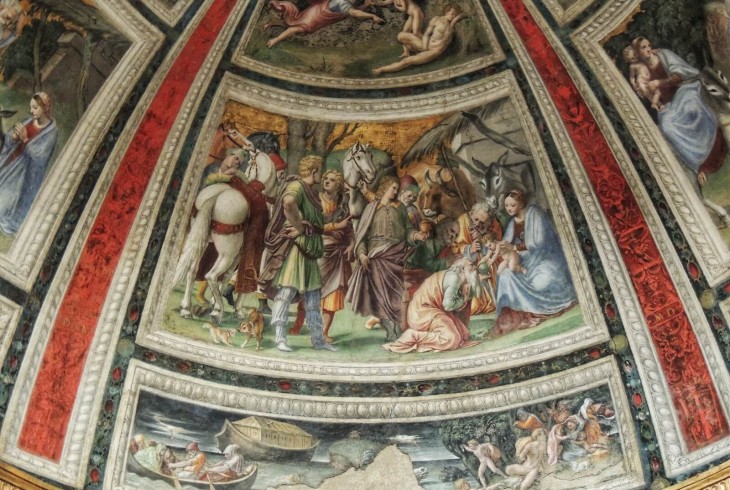This highly detailed color photograph captures an ancient European mural, possibly from a 15th to 17th-century church. The mural, painted on a dome-like ceiling, features multiple interconnected frames. The central frame vividly depicts a very Caucasian representation of the Nativity scene. Here, white and blonde men stand on the ground beside white horses, while a woman in a light blue robe holds a naked baby on the far right. An old man kneels before them, and two other elderly men are present nearby. Included in the scene are a donkey, a bull, and several people apparently praying over the baby. Surrounding frames partially visible in the image depict varied scenes; one shows boats near a shore, another possibly portrays the Garden of Eden with unclothed figures, and others contain indistinct images of people, including a recurring woman in blue. The mural's vibrant colors include blue, red, black, and tan, adding depth and uniqueness to the overall composition.